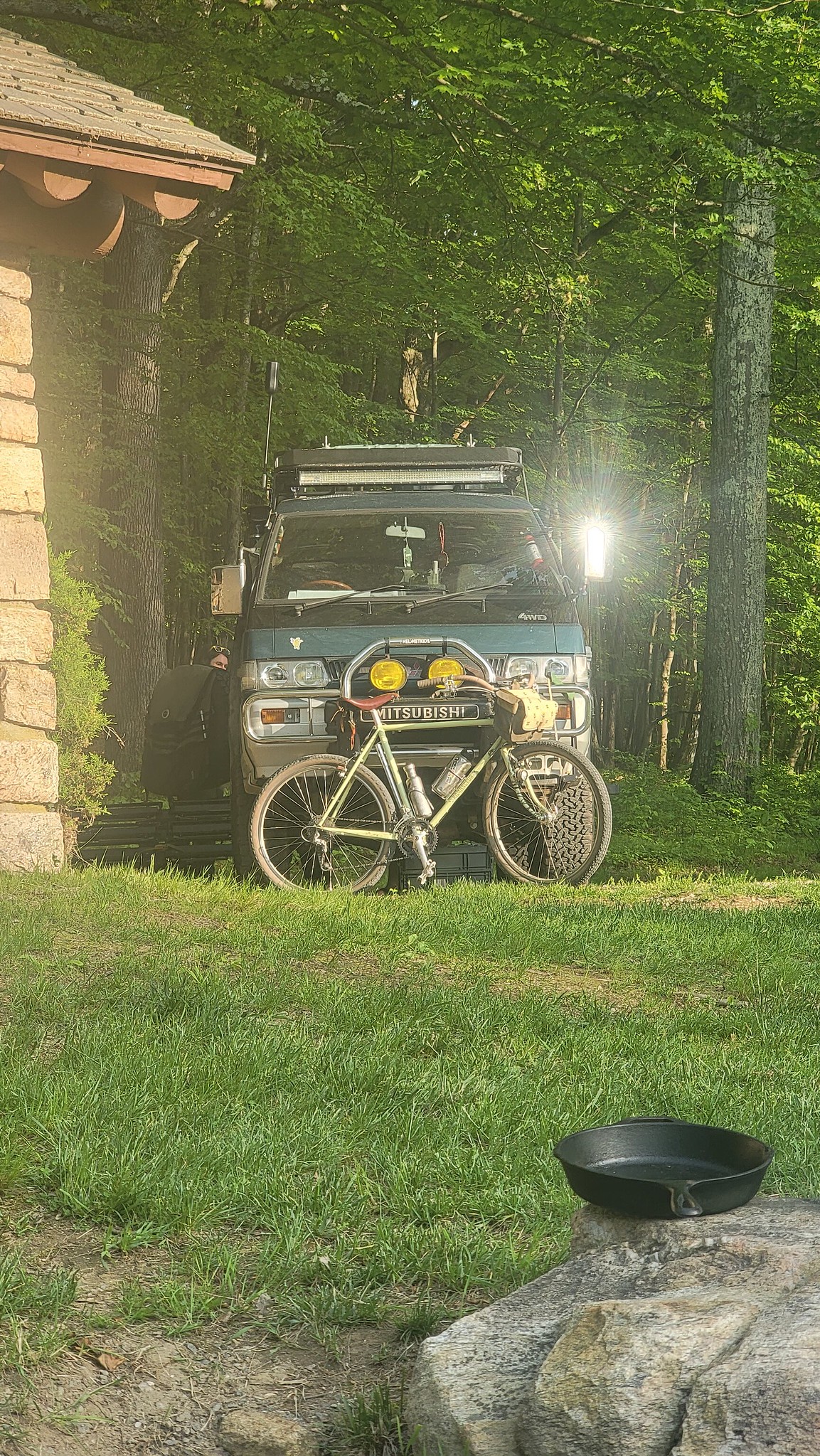The photograph captures a detailed outdoor camping scene set in a grassy area. In the foreground, there's a black cast iron frying pan resting atop a large stone. The middle ground features a green or yellow bicycle with a red seat and black tires, leaning against a light teal or blue Mitsubishi camper van. To the left of the van, part of a brown stone building and its roof are visible. An individual is partially seen near the left side of the vehicle, possibly sitting with a bag or jacket. The background is densely covered with large trees, their trunks and leaves obscuring the sky, contributing to the lush, green ambiance of the setting. The sunlight reflects off one of the camper's side mirrors, adding a touch of brightness to the scene.